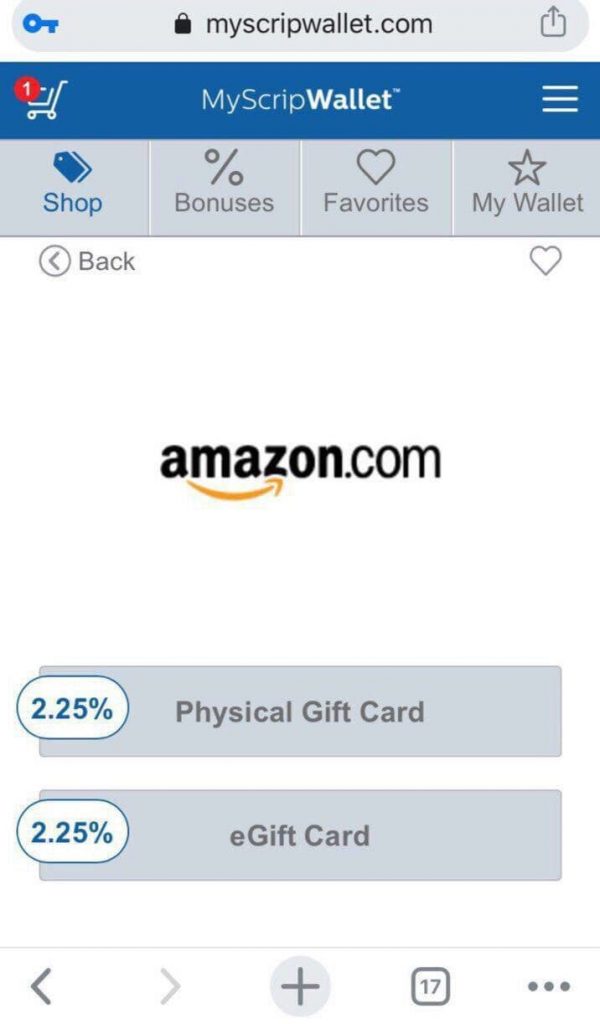A detailed caption of the screenshot from the cell phone displays a mobile web page on MyScripWallet.com. In the address bar, the URL "MyScripWallet.com" is prominently visible, flanked by a blue key icon on the left and a pop-out menu button on the right. The top of the web page features a blue banner with "MyScripWallet" inscribed in white. On the left side of this banner, a shopping cart icon with a red circle and the number "1" indicates one item in the cart. On the right side, the banner shows a three-line dropdown menu button.

Below the banner, the page is divided into four tabs labeled "Shop," "Bonuses," "Favorites," and "MyWallet." The "Shop" tab is highlighted in blue, indicating the active section. Central to the page is the Amazon.com logo accompanied by the iconic smile underneath. Beneath the logo, two gray rectangular buttons labeled "Physical Gift Card" and "eGift Card" are visible. Each button has "2.25%" marked on the left side, likely representing a cashback or discount value. The screenshot also reveals that the user has 17 tabs open in their browser, as indicated at the bottom of the screen.